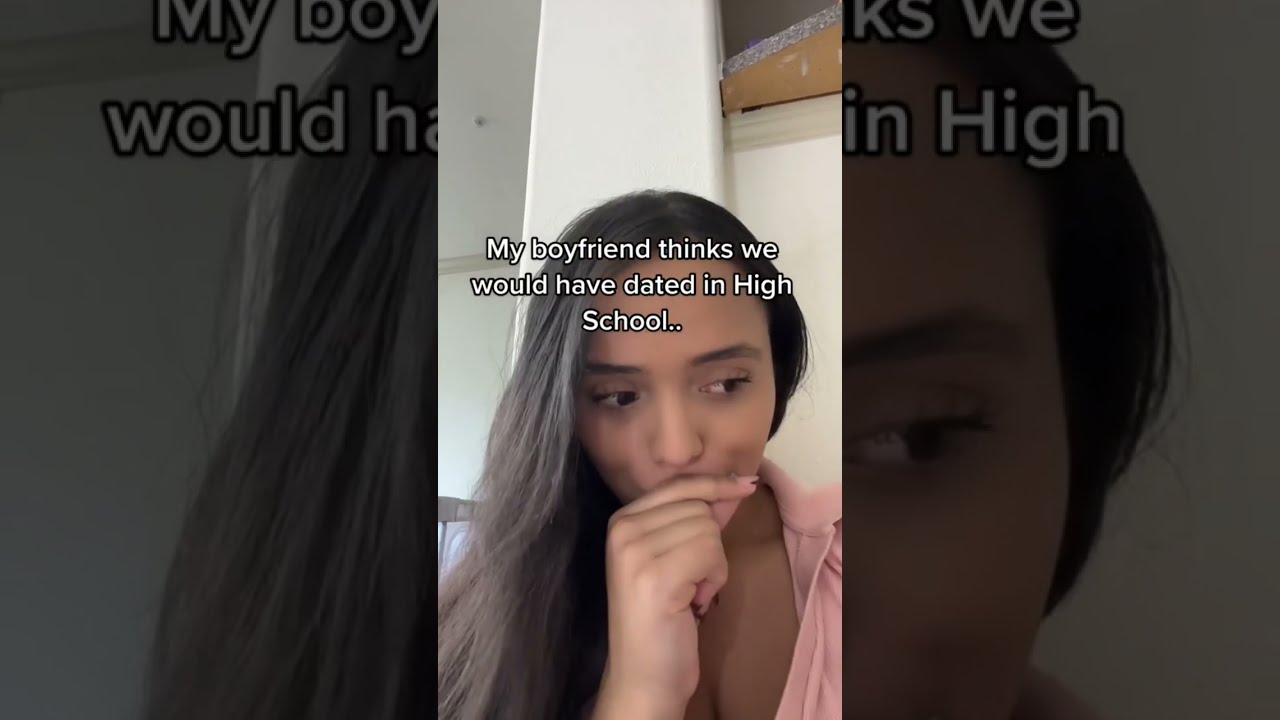In this horizontal, high-definition image, three vertical panels stretch across the width, each capturing portions of the same young woman, creating a layered visual effect. The central focus is a superimposed middle panel, prominently featuring a young woman with long black hair, parted lips, and a pensive expression. Her right hand partially covers her mouth in a contemplative gesture. She is dressed in a pink shirt, her face framed by long eyelashes. 

Directly above her forehead, a line of white text reads, "my boyfriend thinks we would have dated in high school," spanning three lines and succinctly capturing the reflective sentiment. The background is composed of white walls, suggesting a minimalistic indoor space, possibly a bedroom with high ceilings or the illusion thereof due to her seated position.

The left and right panels are darker, blurred close-ups of the same image, drawing attention to the superimposed central portrait. The left panel displays fragments of the text, "my BOY wood HA," partially obscured, while the right panel highlights sections of her face and hair, with visible letters "KSWEI" and "INHI" from the overlapping message. This format, where the central panel resembles a cell phone display taller than it is wide, evokes the aesthetic of social media videos typical of platforms like TikTok or Instagram.